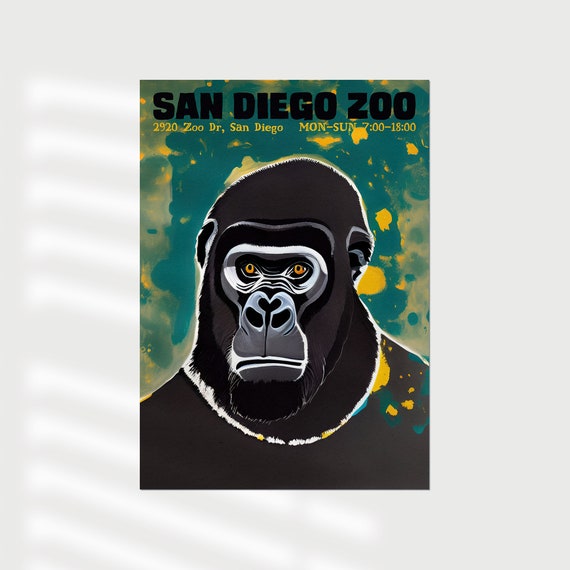This image is a digitally-created illustration of an ape, predominantly showcasing the head and shoulders, set against a white-framed background. The ape is depicted in black, gray, and white tones with golden eyes and accents of white around its eyes. Silver or lighter black hues are noticeable towards its muzzle. Above the ape, large bold black letters read "San Diego Zoo." Below this, in yellow lettering, the text states "2920 Zoo Drive, San Diego, Monday through Sunday, 7 o'clock to 18 o'clock." The background behind the ape features splotches of vibrant teal, light green, yellow, light yellow, and light blue colors. The ape is minimally touched by these colorful blobs, enhancing its contrast against the vivid backdrop. This detailed and engaging design captures attention and emphasizes the zoo's branding and information effectively.